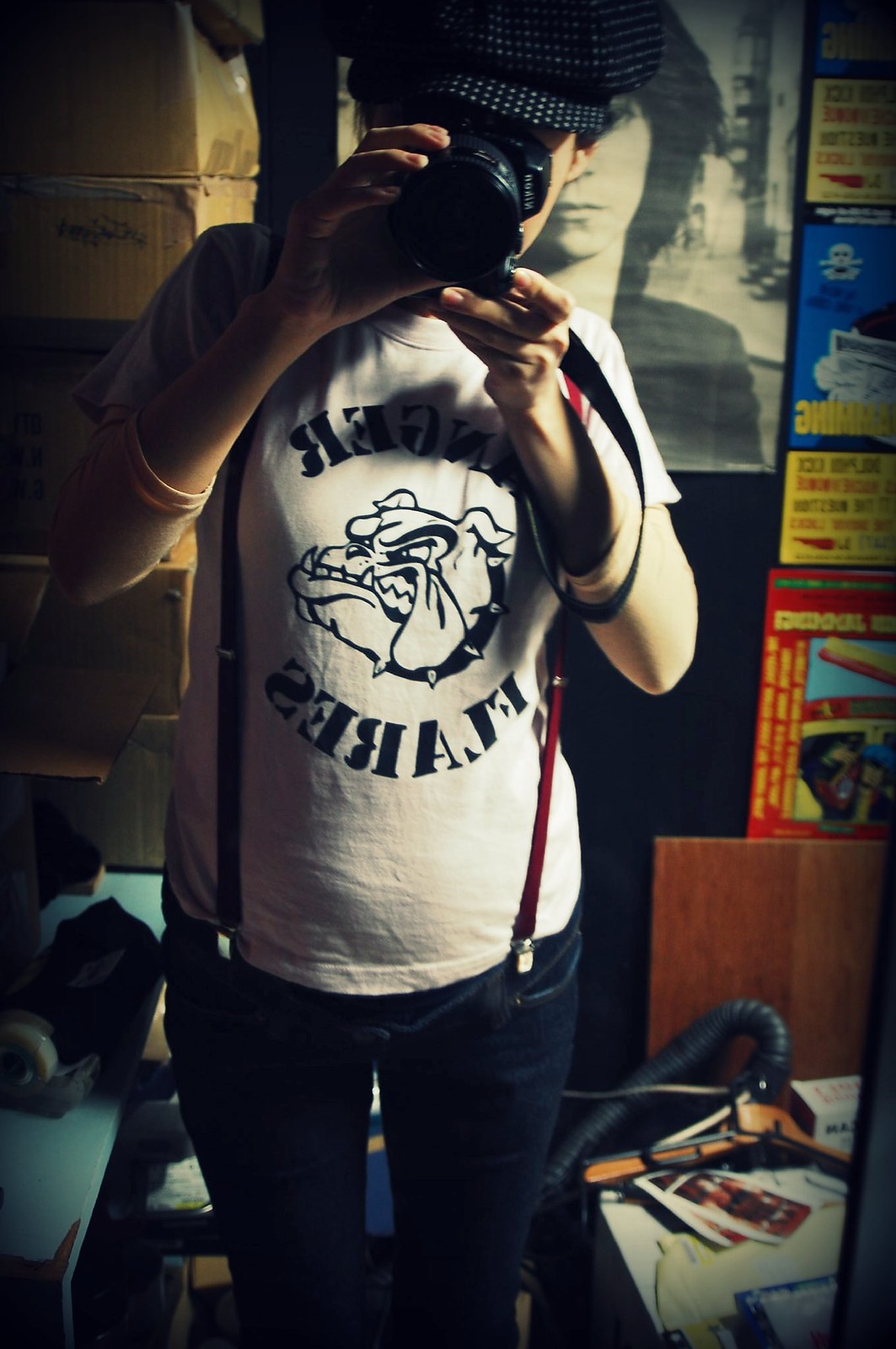The photograph features a man taking a selfie in a mirror using a Nikon camera, possibly a D70. He is wearing a distinct black paperboy hat with polka dots and a white t-shirt adorned with an image of an angry-looking bulldog and the text "Anger Flares" in mirrored writing. Red suspenders are clipped to his dark navy skinny jeans, enhancing his overall hipster, indie, and emo vibe. Behind him, a black and white poster of Jim Morrison hangs on the wall, accompanied by stacks of cardboard boxes. Additional colorful posters with red and yellow writing, along with various items such as a vacuum cleaner or coat hanger, are visible in the room. The light in the room suggests the presence of a window on the right side, as there is no apparent flash in the image.